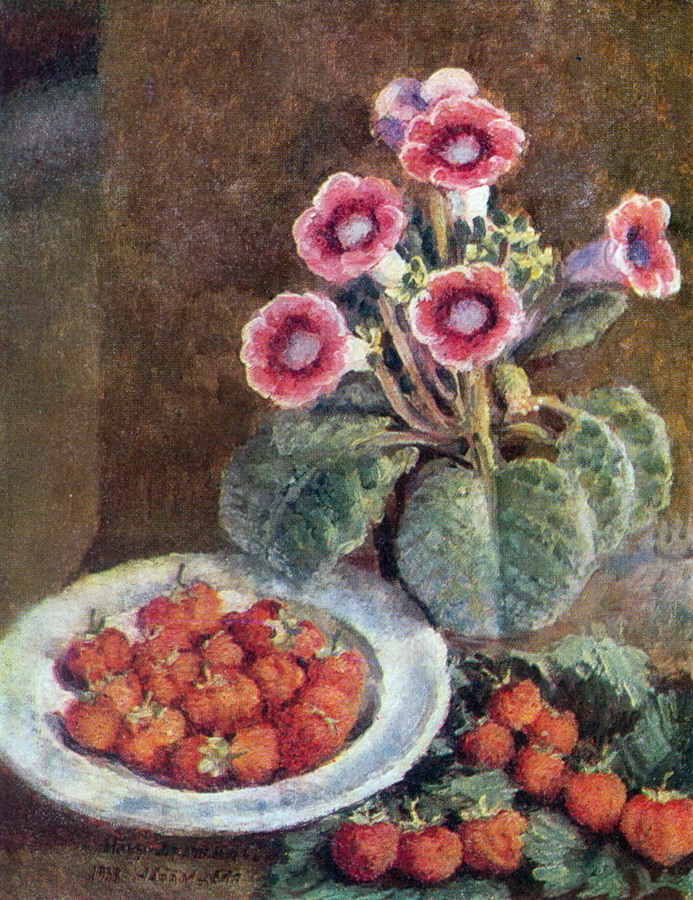This painting features a rustic brown background that sets an earthy tone accented by intricate details. On the right half, a vibrant plant showcases five flowers with a distinctive color pattern: dark pink outer petals, a red ring around the inner petals, and a white center, all supported by brown stems and large, thick green leaves. To the lower left side, a shallow round white bowl holds numerous strawberries with their green stems intact. Adjacent to the bowl, in the lower right foreground, additional strawberries, some still connected to their plants, rest on a bed of green leaves. The brown background and surface extend cohesively across the artwork, enhancing the natural theme. The painting also contains barely noticeable, small, and light writing on the front left side, adding a subtle yet intriguing detail.